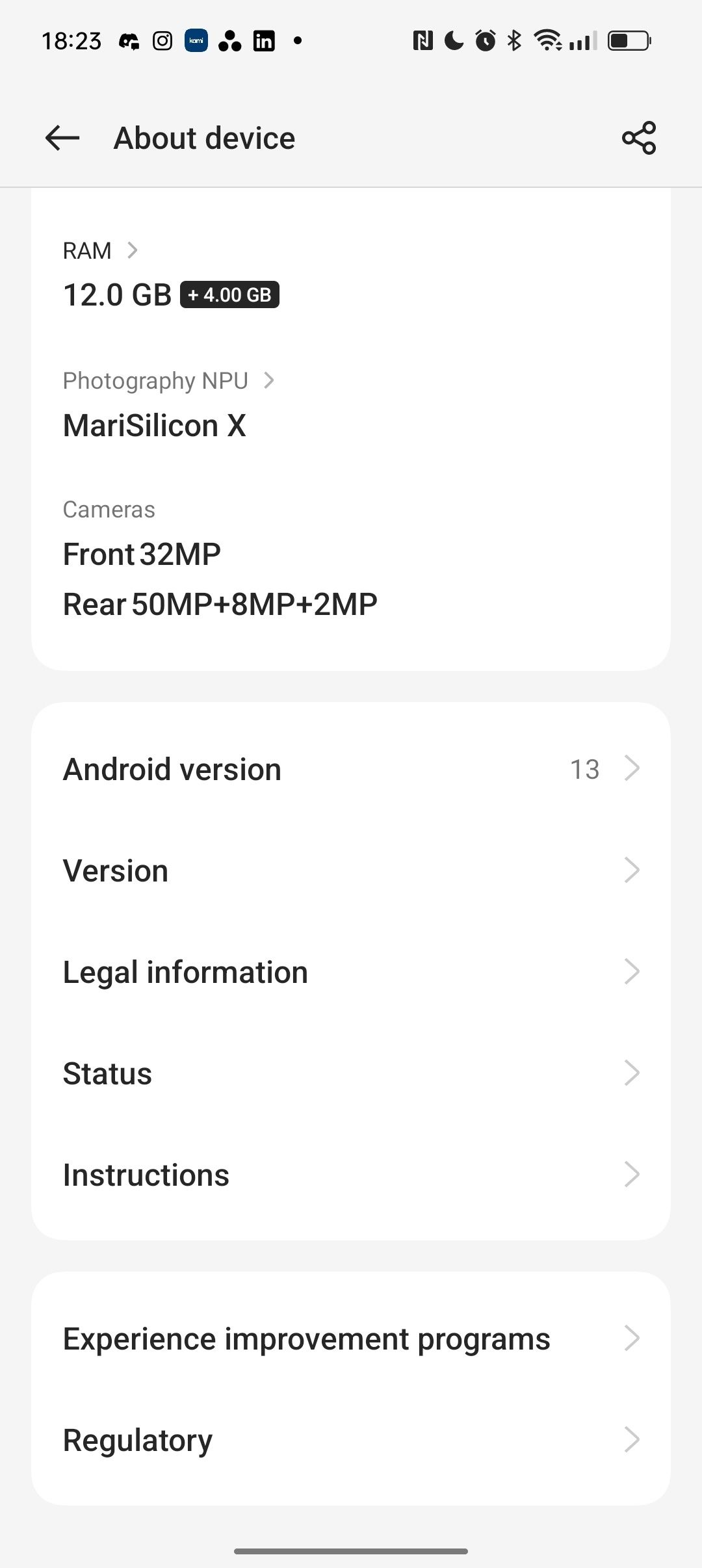A close-up image of a smartphone's settings screen showcases various technical details and system information. At the top of the display, the time is prominently indicated as 18:23, alongside traditional icons for notifications, cellular signal strength, battery life, and Wi-Fi connectivity, all rendered in a standard black color. Below this, the screen delves into more specific device details, including information about the RAM, operating system (Android version), and legal notices. This appears to be a settings interface, providing an array of miscellaneous yet pertinent information about the phone's internal specifications and system status, accessible for users seeking to manage their device or troubleshoot issues.